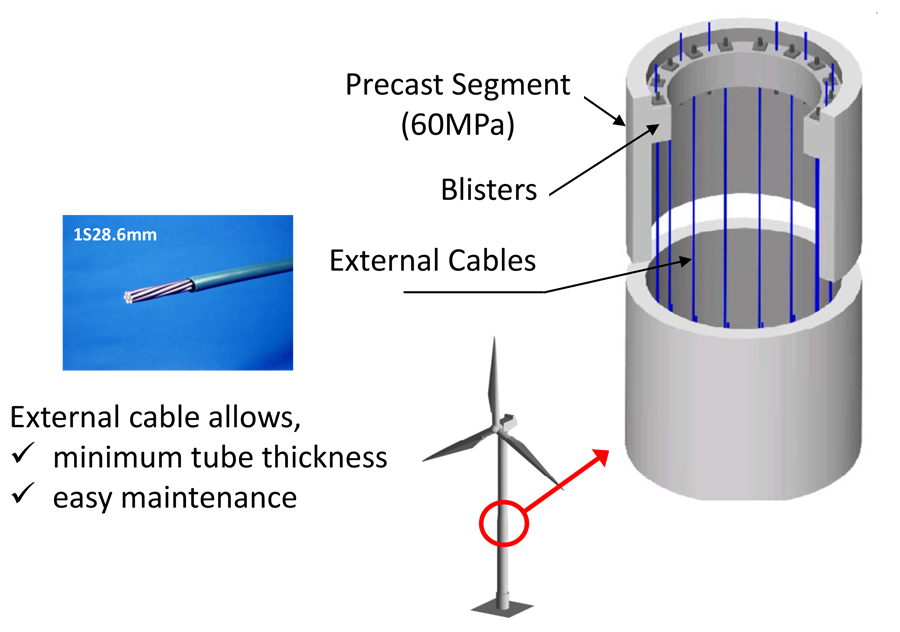This image is an intricate engineer's diagram of the internal cable paths within the vertical mounting post of a three-blade wind turbine. The main focus is a detailed, three-dimensional cutaway view of the cylindrical base, showcasing the internal structure and the arrangement of cables. The cylindrical object is white on the exterior, with blue vertical lines representing the cables running internally from top to bottom. Surrounding the cylinder are blisters and a label indicating "precast segment, 60 MPa," emphasizing the strength and structure of the wall. 

To the left of the cylinder, a close-up of one of these cables is prominently displayed against a blue background. This detailed view highlights the internal components of the cable and includes annotations such as "1s 28.6 mm," suggesting specific measurements, and notes like "external cable allows minimum tube thickness, easy maintenance," underlining the design benefits.

In the bottom middle of the image, there's a smaller depiction of the complete windmill, distinguished by its silver color and mounted atop a vertical post. This smaller diagram is encircled with a red arrow pointing to the larger cutaway view, visually clarifying the relationship between the two sections. This red arrow and circle emphasize the area of the turbine being analyzed in the blow-up diagram, providing context for the internal layout of the cable paths and structural elements.